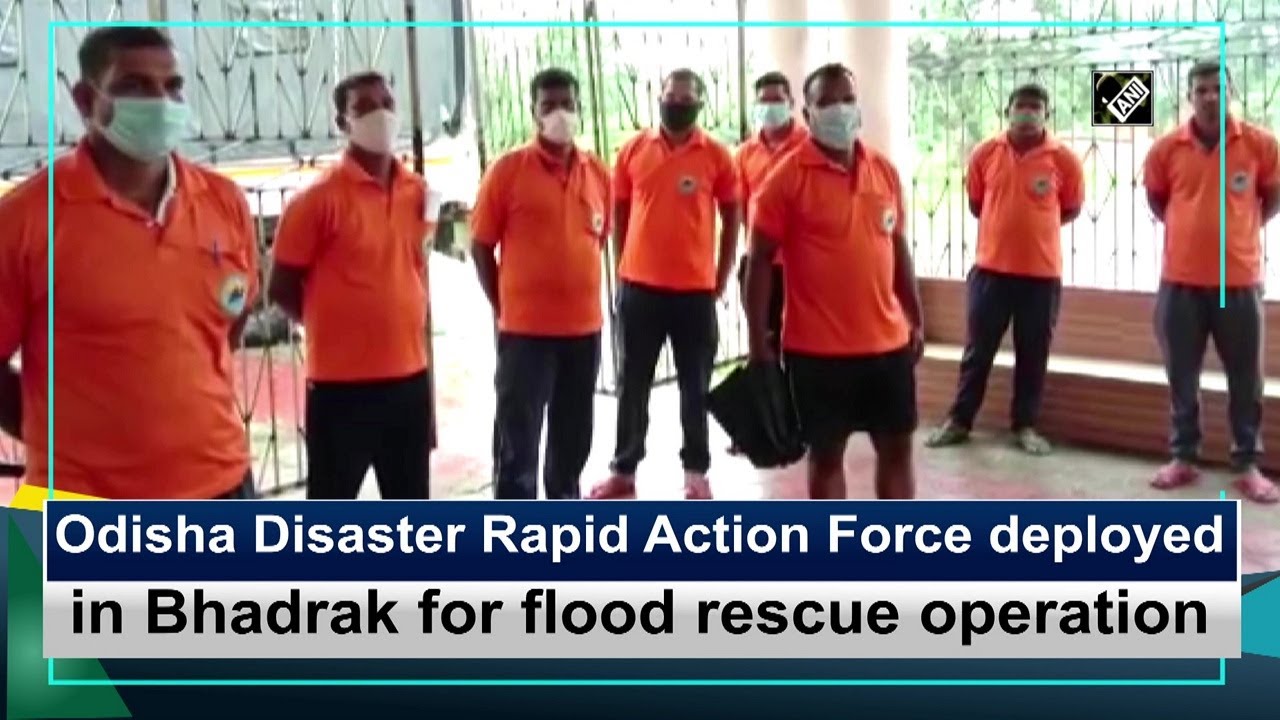The image is a color, landscape-oriented photograph featuring a group of eight men standing side-by-side in an interior space. All are dressed identically in orange polo shirts adorned with emblems on the pockets, black pants, and face masks, with their hands folded behind them, appearing to stand at attention. In the foreground, one man is holding a case. The photograph includes two lines of text at the bottom; the upper line, in white on a dark blue background, reads "Odisha Disaster Rapid Action Force Deployed," and the lower line, in black text on a white strip, reads "in Bhadrak for Flood Rescue Operation." The scene is bordered by an aqua-colored rule, with a black wrought iron gate or fence visible in the background, leading to an outdoor view. The image likely captures the team as they prepare for deployment on a flood rescue mission.